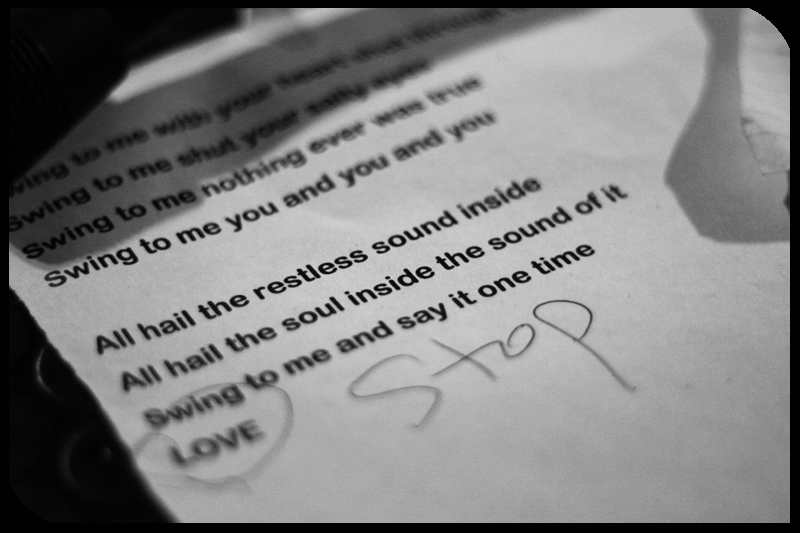This black-and-white photograph, framed with a thick black border, captures a single sheet of paper that appears to contain a poem. The paper rests on a shadowy desk, illuminated to reveal typed text arranged from the top left down to the center and bottom right. The poem includes the lines, "Swing to me, you and you and you," followed by "All hail the restless sound inside, all hail the soul inside the sound of it, swing to me and say at one time, love." Notably, the word "love" is circled in black ink, with "stop" handwritten next to it. The combination of the typed text and the handwritten annotations adds a layer of intrigue to the scene. The photograph is taken at an angle, emphasizing the texture and depth of the paper amidst the monochrome tones.